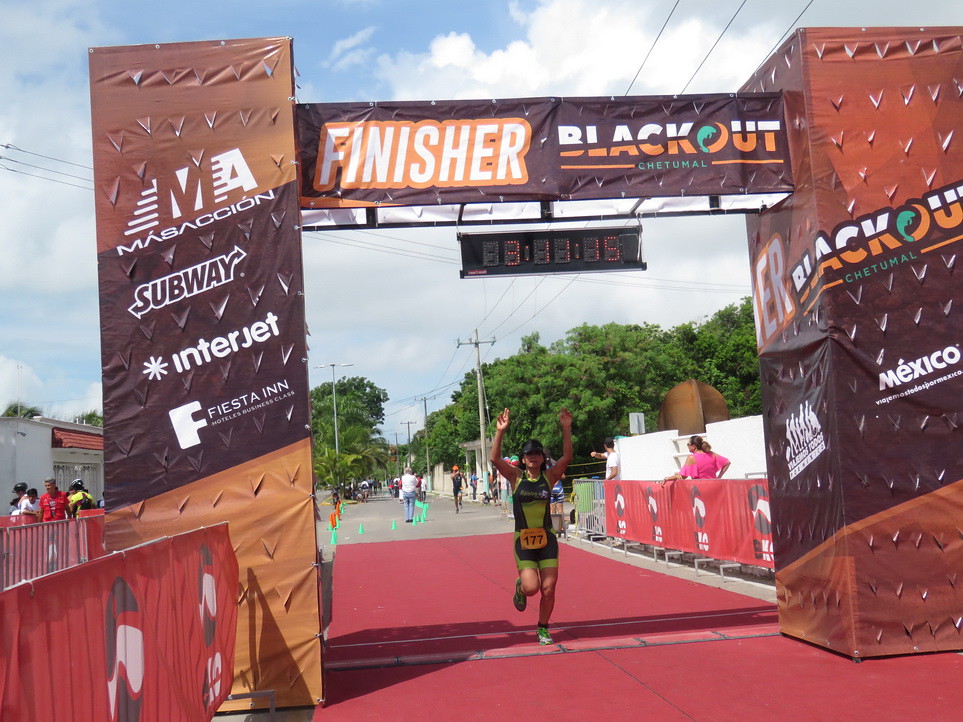In a vibrant outdoor setting on a partly cloudy day, a photograph captures the triumphant moment of a woman of Latino descent crossing the finish line in a race, possibly a marathon or triathlon. She exudes energy and accomplishment, her arms raised high above her head. She is dressed in a striking black and fluorescent green tank top and matching shorts, donning green and white sneakers and a black visor. The number '177' is prominently displayed on her waist. 

The finish line is a visually imposing structure with two light brown columns adorned with logos from various sponsors, such as Subway, Interjet, and Fiesta Inn, all wrapped in plastic paper. A large banner spans the columns, displaying the text "FINISHER BLACKOUT CHETUMAL" prominently at the top. Just beneath the banner, a digital clock ticks away, showing her finish time as 3:11:15. She sprints across a vivid red carpet laid out beneath the finish line, adding to the dynamic energy of the scene. Spectators are lined along the street, witnessing her moment of victory, adding to the sense of communal celebration.